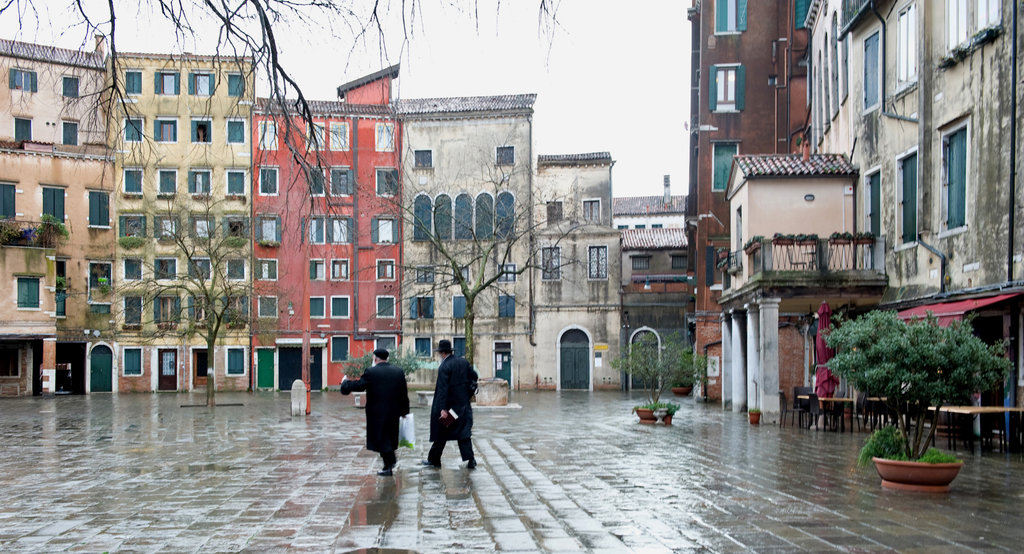The photograph captures a rainy day in a city courtyard, likely the Jewish Ghetto in Venice. Two men, central to the image, are walking across a wet, rectangular stone-paved square. They are dressed in dark attire: long black trench coats, black dress pants, and black shoes. Each man wears a black hat; the man on the right sports a fedora, while the man on the left dons a newsboy cap and carries a white plastic bag.

Surrounding the courtyard are multi-storied stone buildings painted in various colors, adding a vibrant backdrop. On the left, the buildings transition from orange at the bottom to tan at the top, followed by a yellow building, a red building, a gray building, a white building, and another gray building. The buildings on the right continue this colorful array.

Many of these buildings feature balconies adorned with plants, indicative of daily life and residential character. Some trees in the square are leafless, perhaps indicating the season. Red potted plants with green leaves add splashes of color to the courtyard. Among the white buildings on the right, one appears to be an old hotel, distinguished by its pillars and aged gray facade. The architectural details in the image, such as arched windows and doorways, contribute to the historic atmosphere of the scene.